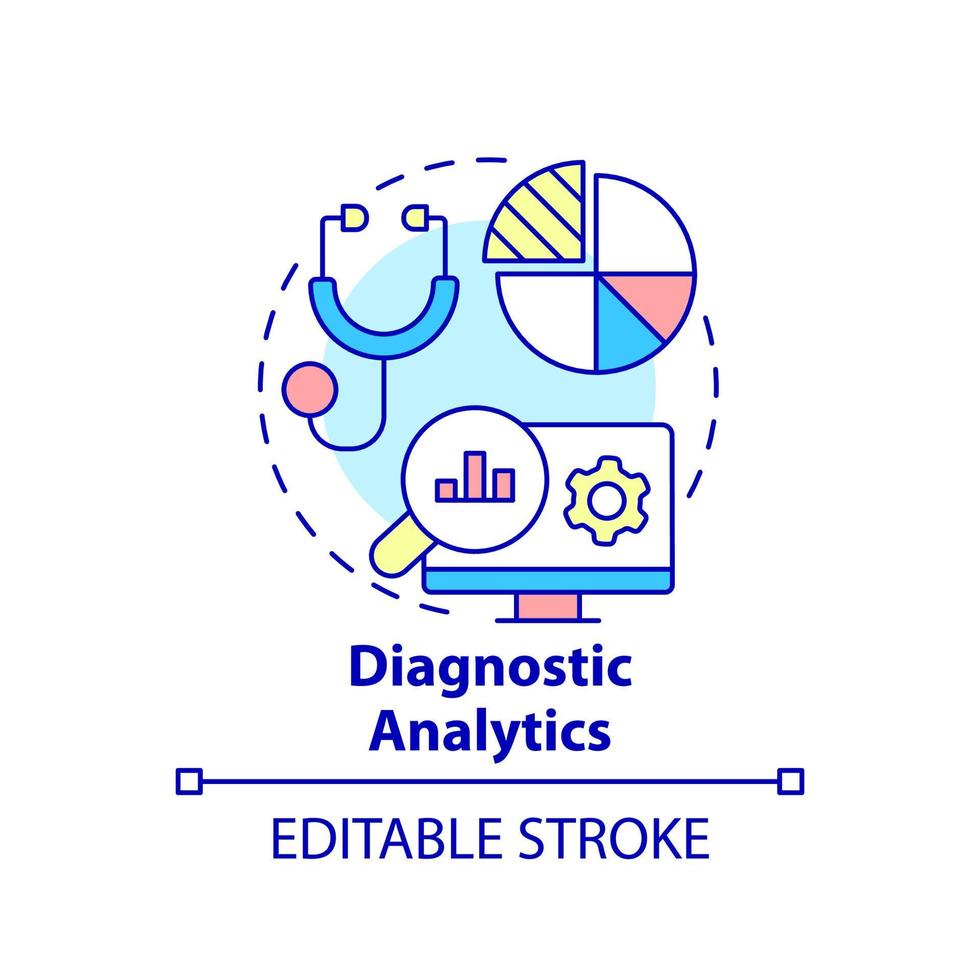The image features a central light blue filled circle encompassed by a dotted circular line on a white background. This image, designed in a clip art style reminiscent of a medical brochure, is likely intended for a doctor's office or hospital use and possibly even for a medical textbook. Surrounding the central blue circle are various medical and analytical icons, including a stylized stethoscope with yellow earpieces, a pink diaphragm, and a blue tube. Adjacent to it is a pie chart with segments in white, pink, blue, and yellow, with the latter segment lifted out and detailed with dark blue stripes. Another icon shows a computer screen with a yellow gear on the display, a blue base, and a pink pedestal. In front of the computer screen is a circular icon featuring a pink bar graph outlined in dark blue. Below these shapes, the bold blue text reads "Diagnostic Analytics," with a small blue separating line underneath, followed by the text "Editable Stroke."